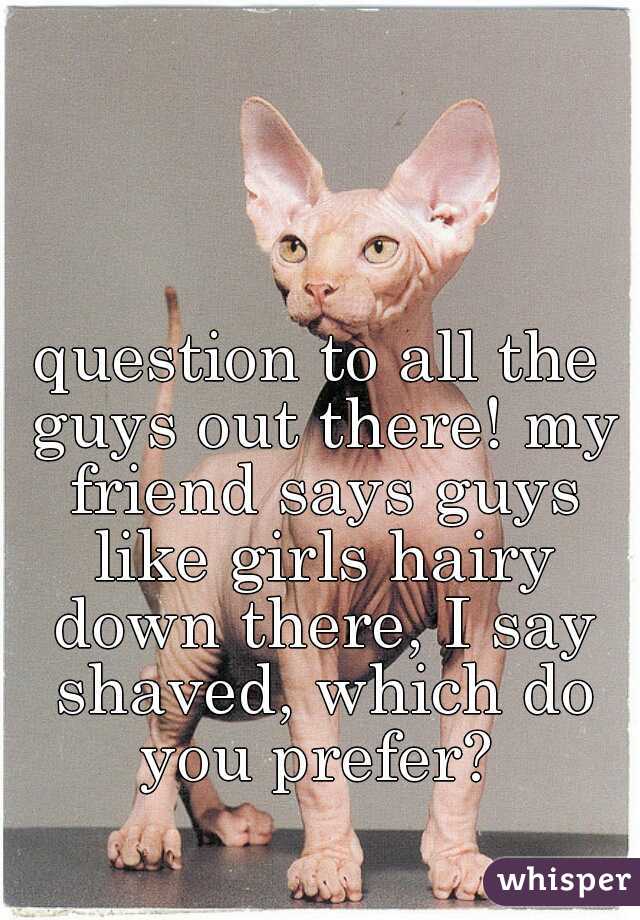The image is a provocative meme featuring a hairless cat, likely a Sphynx breed, standing prominently on a dark gray surface. The cat, which is bald and has large ears, appears in front of a plain, light gray background. Overlaid on the image is white text in a stylized, all-lowercase font that reads, "question to all the guys out there! my friend says guys like girls hairy down there, i say shaved. which do you prefer?" At the bottom right-hand corner, there is a tag with the word "whisper" in white text on a purple background, indicating this is likely a post from a social media platform designed to spark discussion.